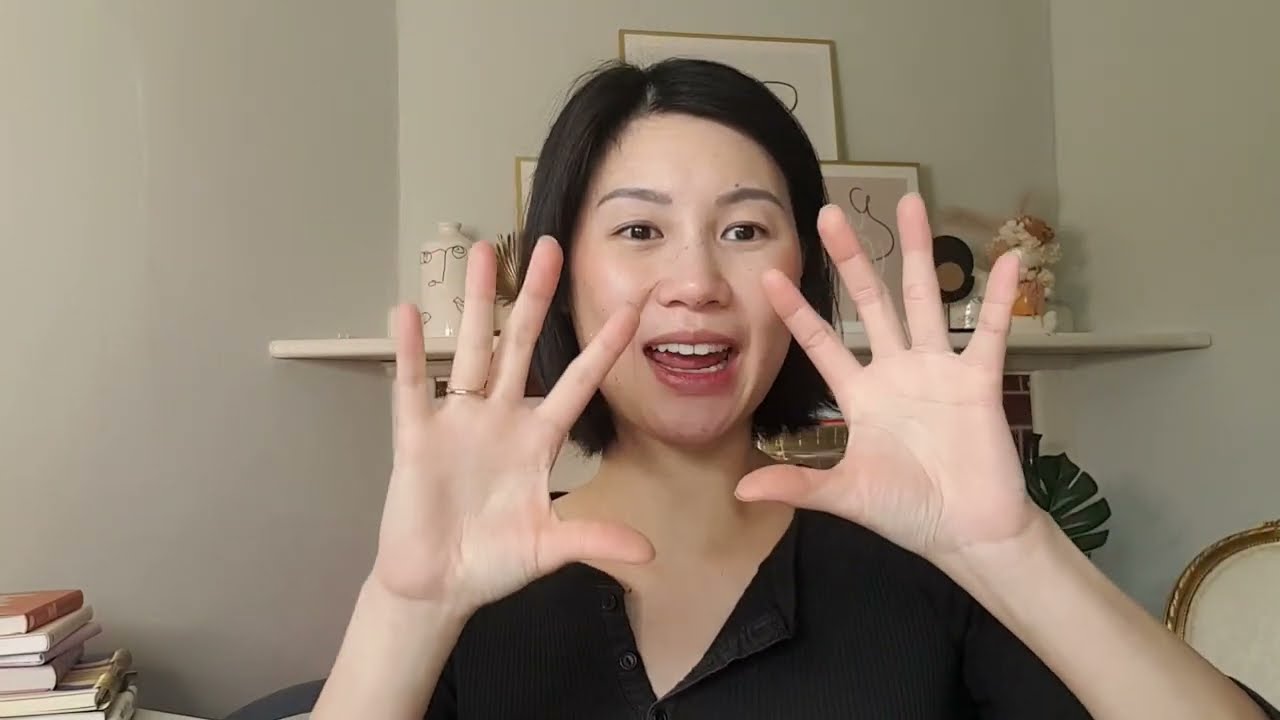The image features an Asian woman prominently, with short black hair and styled eyebrows. She is sitting in a room with monotone off-white walls, reminiscent of a residential bedroom. Her hands are raised up high by her face, with her fingers spread apart and her palms facing the camera. The woman appears to be either surprised or speaking, as her mouth is slightly open, revealing her white teeth and her tongue. She is dressed in a black collared shirt, which is partially unbuttoned at the top. To the right of the woman, a table with several books is visible, while to her left, part of a chair can be seen. Behind her, there is a shelf mounted on the wall, adorned with various knick-knacks, including framed pictures, artwork, ceramic figures, and a faux plant. Additionally, a portion of what appears to be a brick wall or fireplace is also visible directly behind her. A ring is noticeable on her right ring finger, suggesting she may be married. The woman takes up most of the frame, capturing a dynamic moment as if she's in mid-conversation or performance.